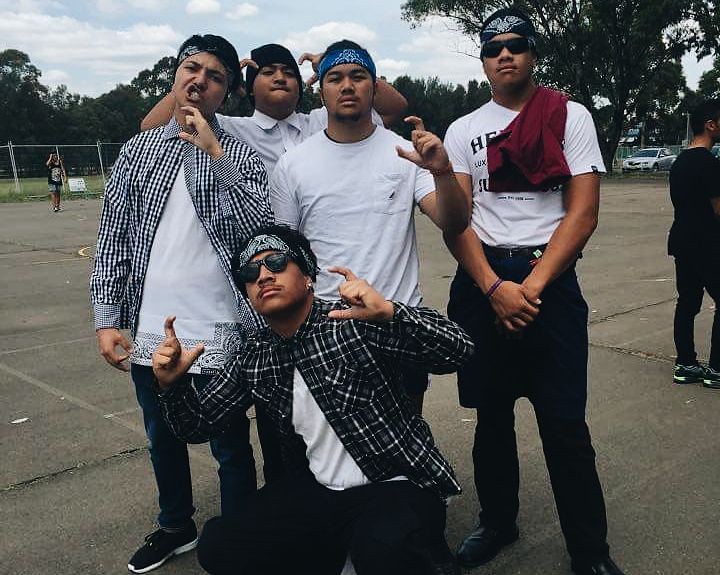This photograph captures five young men, likely in their late teens or early twenties, posed together at what appears to be a public park or playground. All five are dressed in white t-shirts, with two of them wearing black and white plaid shirts over their t-shirts. Four of the men sport headbands while the fifth wears a black stretch cap. One young man is kneeling in front of the group, wearing sunglasses and making a hand gesture, a C shape formed with his thumb and forefinger, which might indicate group affiliation. Another individual on the right also has his hands clasped in front of him. The setting includes a tree line in the background, additional people using the playground, a chain-link fence on the left, a car parked in the distance, and an asphalt paved surface, possibly a basketball court. The overall vibe suggests a moment of camaraderie and playful posing.